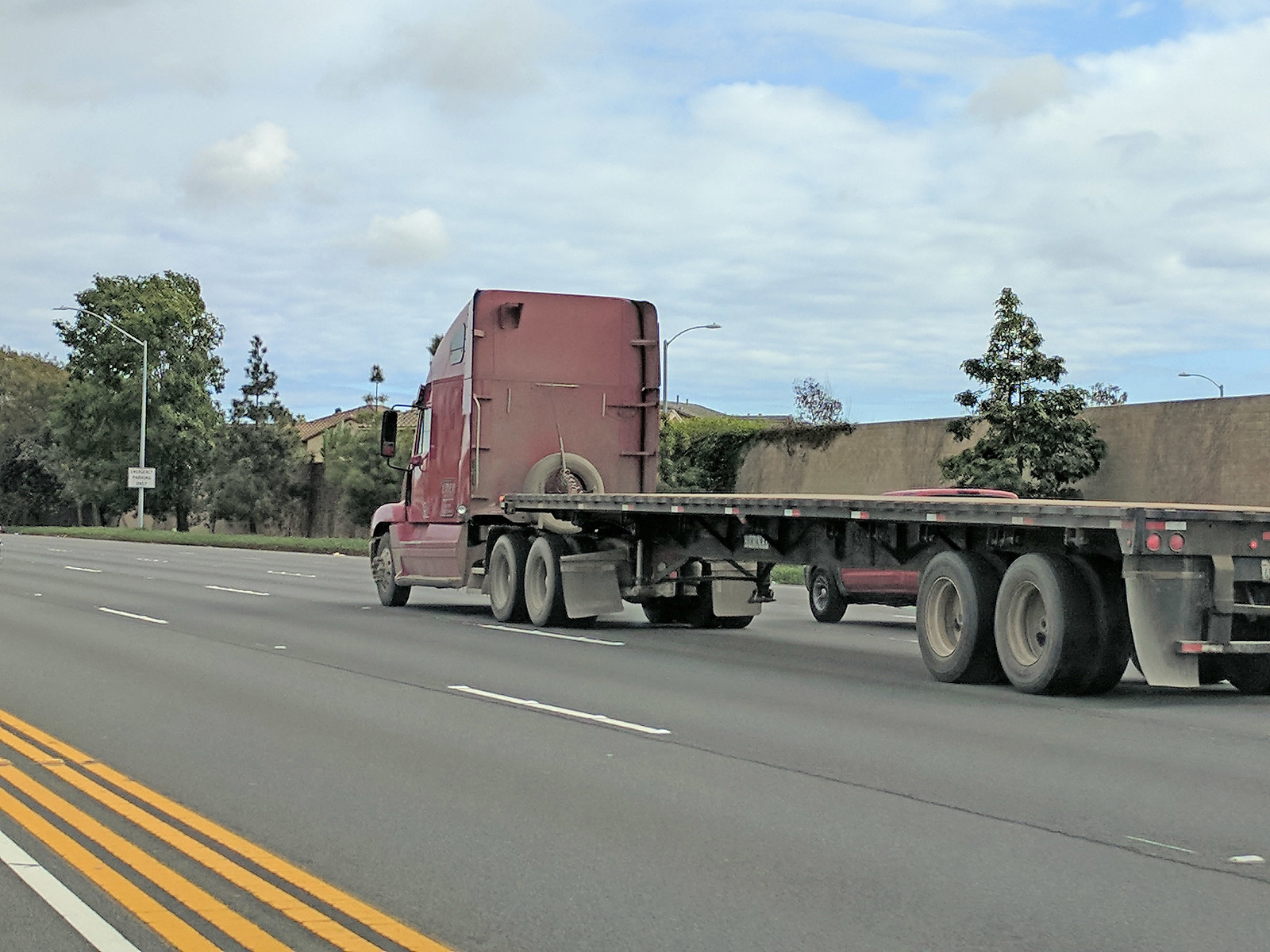This detailed photograph captures a large red-cab semi-trailer truck with an empty flatbed, driving on a multi-lane highway. The image is remarkably clear, showcasing the semi-truck's five wheels visible on the left side and four on the right. The truck is moving quickly, as suggested by its crisp depiction despite being in motion. Positioned in the third lane from the right, the truck is flanked by a partially obscured red pickup truck in the fourth lane. The highway features distinct road markings, including white dashed lines and groups of yellow lines, indicating lane divisions and median separation.

In the background, a mix of greenery and infrastructure is visible. A bank of green trees lines the left side, while a large concrete wall stretches across the highway's far side, topped by more trees. Adding to the scene's complexity are several streetlights and residential houses with tiled roofs peeking above the wall. The sky overhead is overcast, providing a muted blue-gray backdrop that emphasizes the vivid colors of the vehicles below. Notably, a face is discernible in the truck's rearview mirror, adding a subtle human element to the dynamic scene.